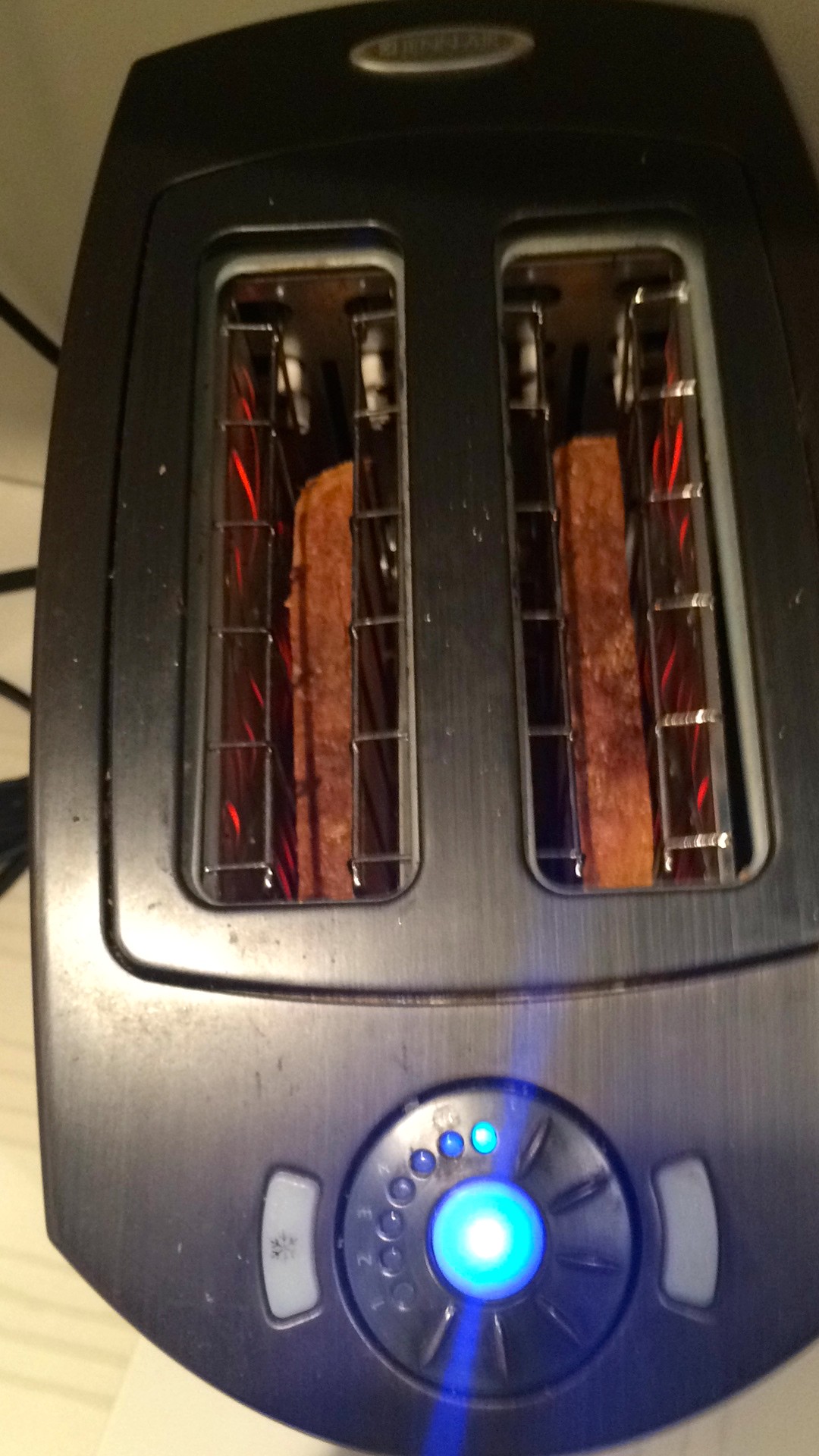In this top-down view of a modern, dark gray toaster, we can see it toasting two slices of thin, darkening bread that appear almost ready. The toaster features a distinctly bright blue button in the center of its control panel, surrounded by various smaller buttons and settings likely used to adjust the toast's darkness level, which seems to go up to seven. The blue button is flanked by two almost dull gray buttons, one of which appears to have a snowflake symbol on it. The illuminated red wires inside clearly indicate that the toaster is on. The toaster is built to hold just two slices, suggesting it’s a compact, single-task machine ideal for limited counter space. The toaster rests on a tabletop with no visible text or branding in the image.